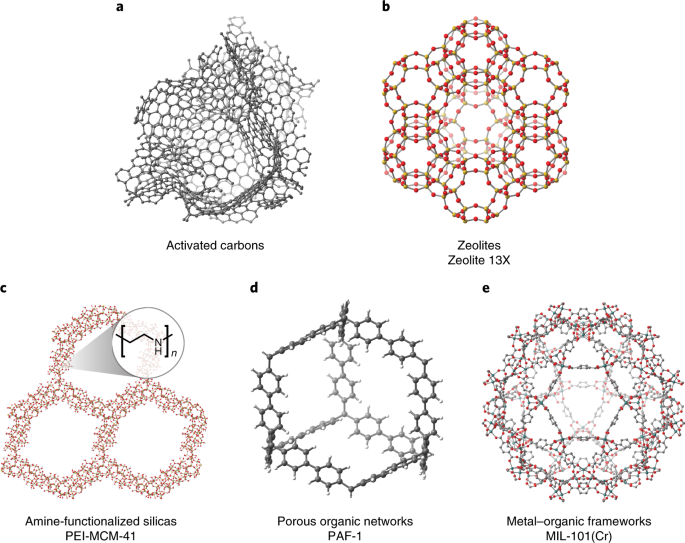The image presents detailed diagrams of five types of chemical structures, labeled A through E, each accompanied by descriptive labels. At the top, Structure A features a black and white depiction of interconnected items labeled "activated carbons." To its right, Structure B displays multiple stop sign-like shapes grouped together, labeled "zeolites, zeolite 13X." On the bottom row, to the left, Structure C showcases three circles with a close-up inset highlighting a black circle on top of one of them, along with the letters N, H, and N, labeled "amine functionalized silicas, PEI-MCM-41." In the middle, Structure D is a black and white arrangement labeled "porous organic networks, PAF-1." Finally, on the right, Structure E consists of red and gray dots and lines, indicating "metal-organic frameworks, MIL-101 (Cr)." The background of the image is white, providing a clear contrast for the colorful and detailed chemical diagrams.